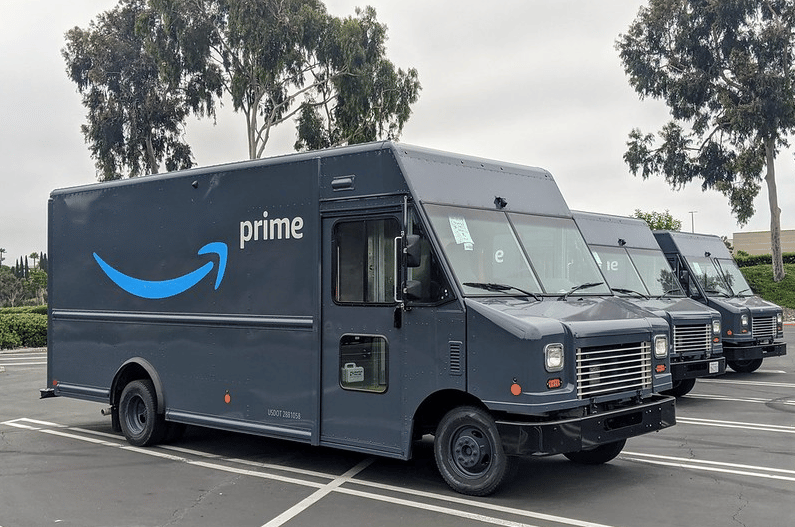In this color photograph, we see a trio of Amazon delivery vans lined up on a multi-lane street, emphasizing the logistics network in action. The vans are distinctly gray, and only the full side profile of the van on the left is fully visible. This van prominently displays the word "Prime" in white font, accompanied by Amazon's iconic blue smile logo that incorporates a checkmark design. Above, the sky is overcast, signaling a gray, cloudy day. Flanking the street are a couple of shade trees, with one particularly tall and slender trunk visible on the right side of the image. In the background, there appears to be a beige building, possibly part of a strip mall. The bottom left corner reveals a small portion of the asphalt street, grounding the scene in an urban setting.